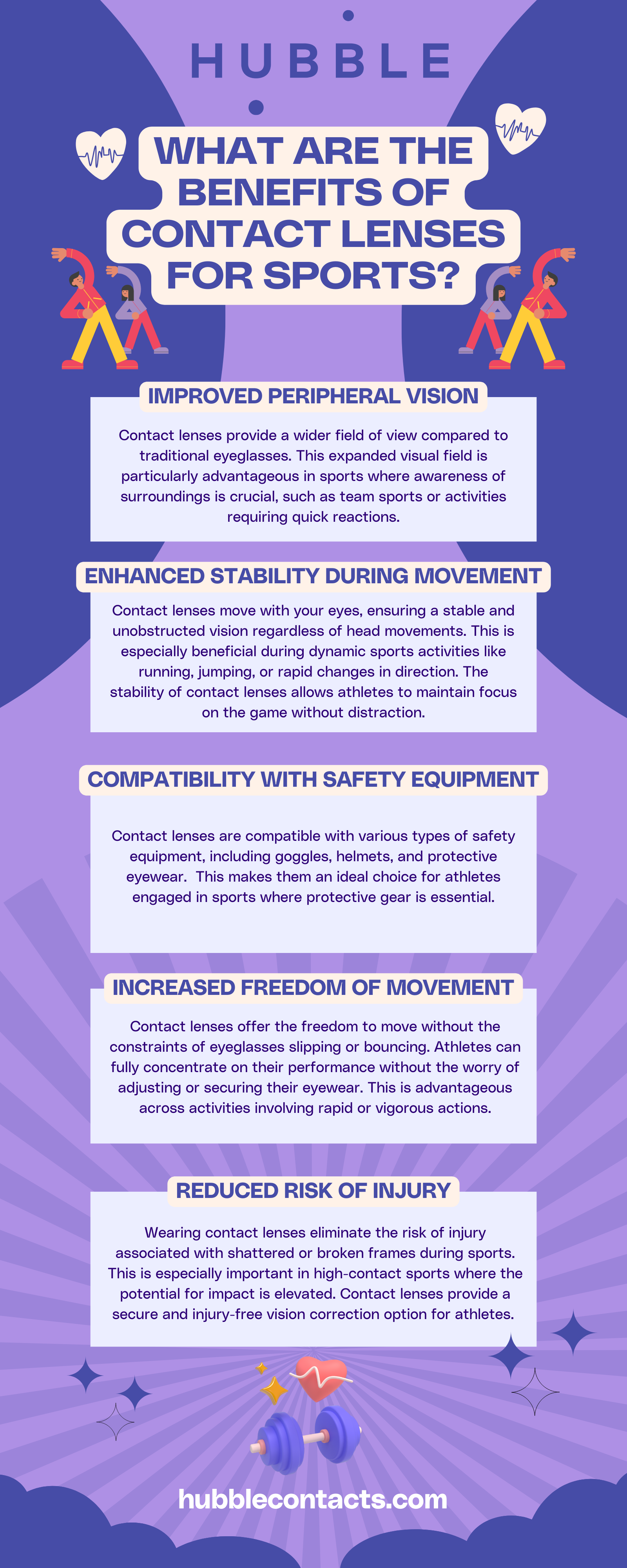An advertisement and informational sheet for Hubble Contacts is meticulously presented on a piece of paper adorned with two shades of purple: light purple and dark purple. At the top, the name "Hubble" stands out in bold, capitalized purple letters. Below, in crisp white text, the headline poses a compelling question: "What are the benefits of contact lenses for sports?"

The visual layout features two sets of individuals performing stretches, with two people positioned on the left and two on the right, symbolizing athletic engagement. Centrally located on the page is a detailed list of benefits that highlight why contact lenses are advantageous for sports enthusiasts:

1. **Improved Peripheral Vision**: Contact lenses allow for a wider field of vision compared to glasses, ensuring athletes can better monitor their surroundings.
2. **Enhanced Stability During Movement**: Unlike glasses, contact lenses stay in place regardless of rapid movements, providing consistent, clear vision.
3. **Compatibility with Safety Equipment**: Contact lenses are seamlessly compatible with helmets and other protective gear, eliminating the hassle of adjusting eyewear.
4. **Increased Freedom of Movement**: Without the constraint of frames, athletes enjoy a fuller range of motion.
5. **Reduced Risk of Injury**: Contacts don't break or shatter, reducing the risk of injury from broken lenses during physical activities.

Each benefit is accompanied by a couple of sentences elaborating on its specific advantages, offering a comprehensive understanding for the reader. At the bottom of the sheet is the company's website, hubblecontacts.com, for further information.